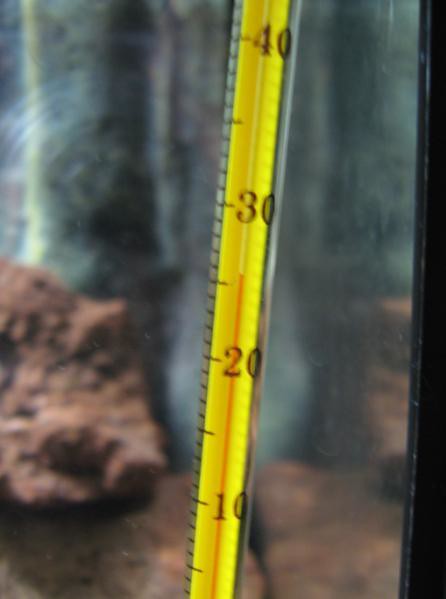A detailed close-up photo features a yellow, slender thermometer with a blurred, silvery reflective backdrop that suggests a potentially rocky or metallic surface. The backdrop, scattered with white streaks and scratch marks, reflects a brownish hue reminiscent of a rock. The thermometer display starts at 10 and extends up to 40 with small black dashes marking each unit. The mercury level is visible just above the halfway dash between 20 and 30, indicating a precise temperature of approximately 26 degrees. The measurement scale—whether Fahrenheit or Celsius—is unspecified.